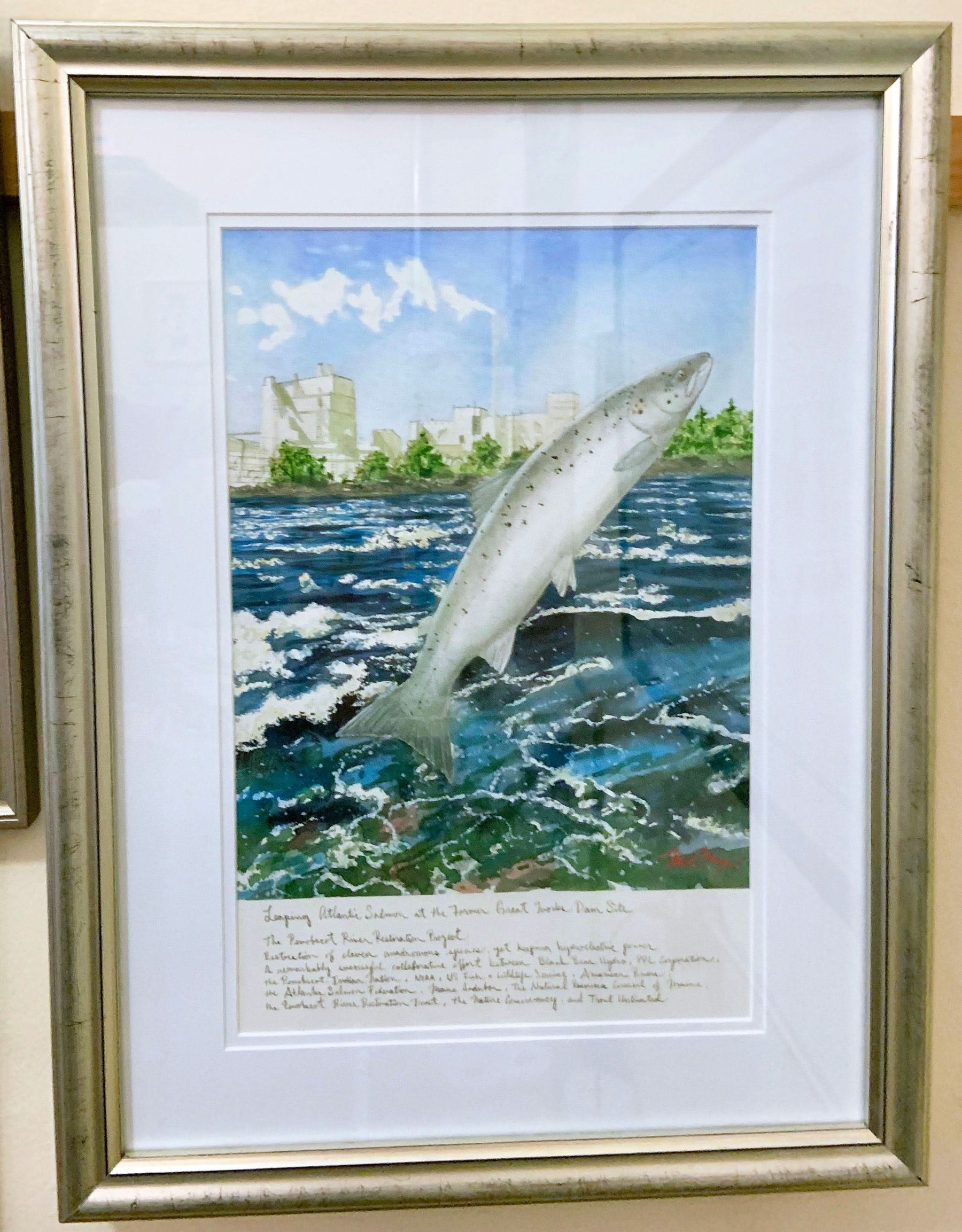The image features a striking depiction of an Atlantic salmon mid-leap, emerging from turbulent, dark blue waters accented with shades of sea foam green. The water splashes energize the scene, indicating a strong current. The salmon itself is solid gray with white markings and spots, showcasing its strength and grace. In the background, hand-drawn, antiquated buildings and scattered trees stand under a sky where a few white clouds float. The bottom quarter of the image contains a handwritten description in cursive script, offering context about the scene. The artwork is surrounded by a matted white border and encased in a gold frame that appears slightly tarnished. The entire piece hangs on a beige wall, positioned next to another picture, suggesting it is part of a larger display. The frame casts subtle shadows, hinting at its interaction with surrounding elements and light sources. The detailed, almost lithographic quality of the image evokes a sense of nostalgia and artistry.